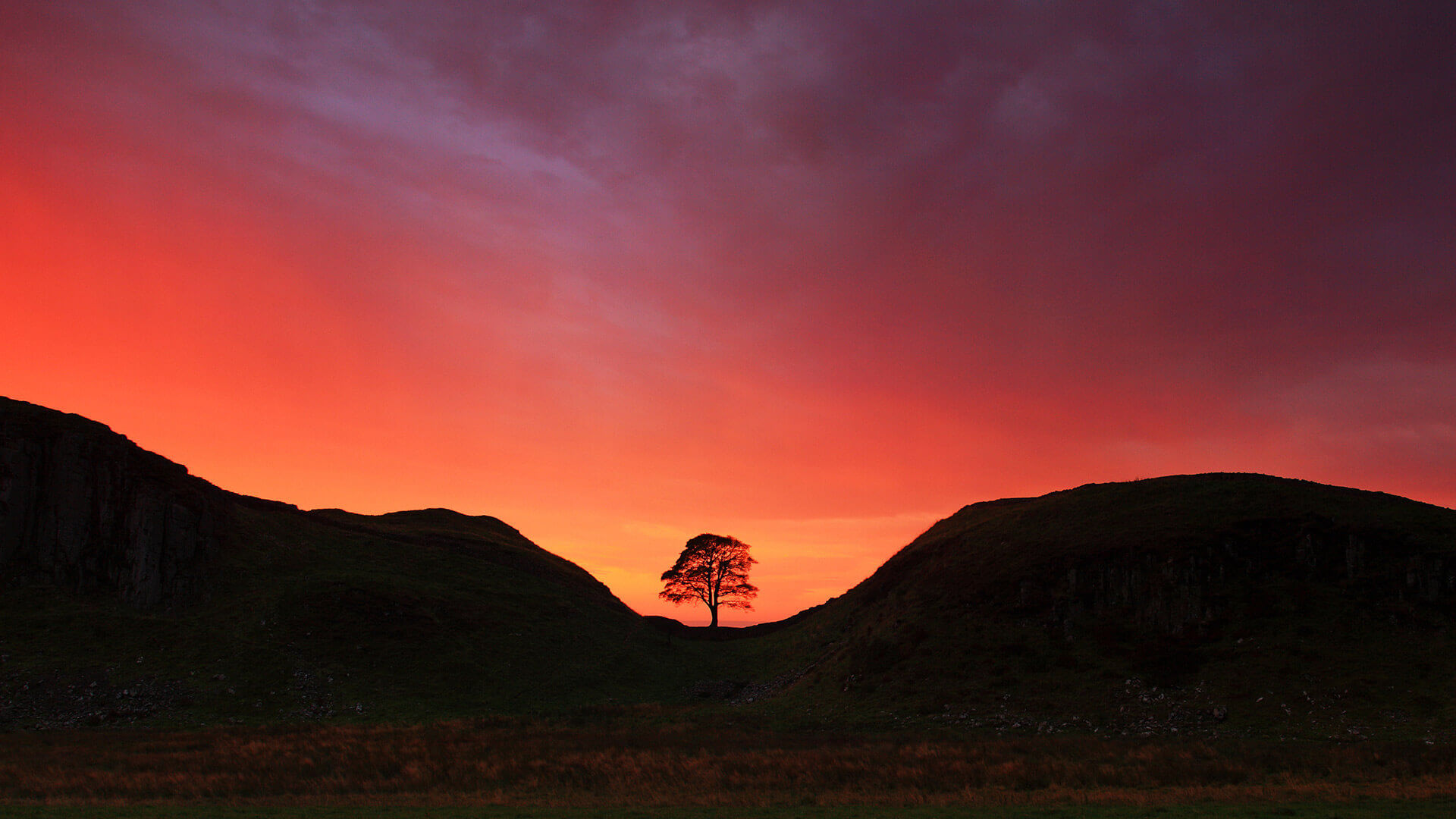The photograph captures a striking image of a lone tree at dusk, framed against a vibrant sky painted with hues of red, burgundy, orange, and yellow. The tree, devoid of any surrounding vegetation and centrally positioned, stands between two black-colored hills, creating a stark silhouette against the dramatic sunset backdrop. The hill on the right is flatter compared to the one on the left, which features two distinct peaks. The fiery sunset light illuminates the tree from behind, casting its leaves in a red hue and bathing the surrounding grass or vegetation at the base in a similar warm tint. The sky, intensely vibrant near the horizon with fire orange shades, transitions to a darker, grayer tone as it extends upward, enhancing the overall dramatic effect of the scene. This visually compelling image leaves a lasting impression with its brilliant colors and the stark contrast of the solitary tree against the undulating landscape.